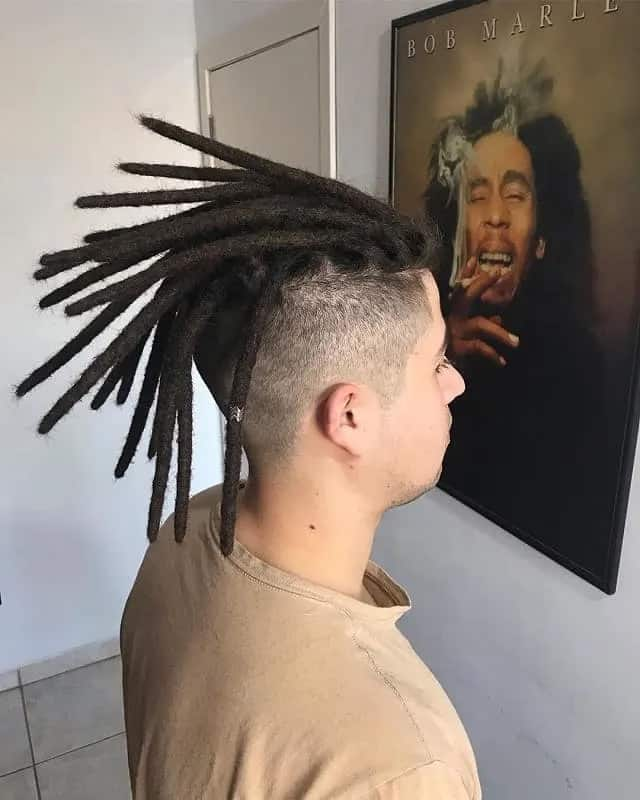A young man, likely in his early teens, stands in front of a white wall adorned with a Bob Marley poster. He wears a plain brown shirt and his hair is styled into a unique dreadlock mohawk, where the sides of his head are shaved, leaving long dreadlocks that extend to his shoulders. These dreadlocks, some adorned with small metal rings, frame his face with scruffy facial hair. The poster on the wall features Bob Marley with an afro, holding a cigarette in his right hand, with smoke curling up above his face and into his hair. The setting appears to be indoors, possibly an art studio or a hallway in a house, indicated by the white walls, white door, and laminate tile flooring. The young man stands in profile, intensely gazing at the iconic image of Marley.